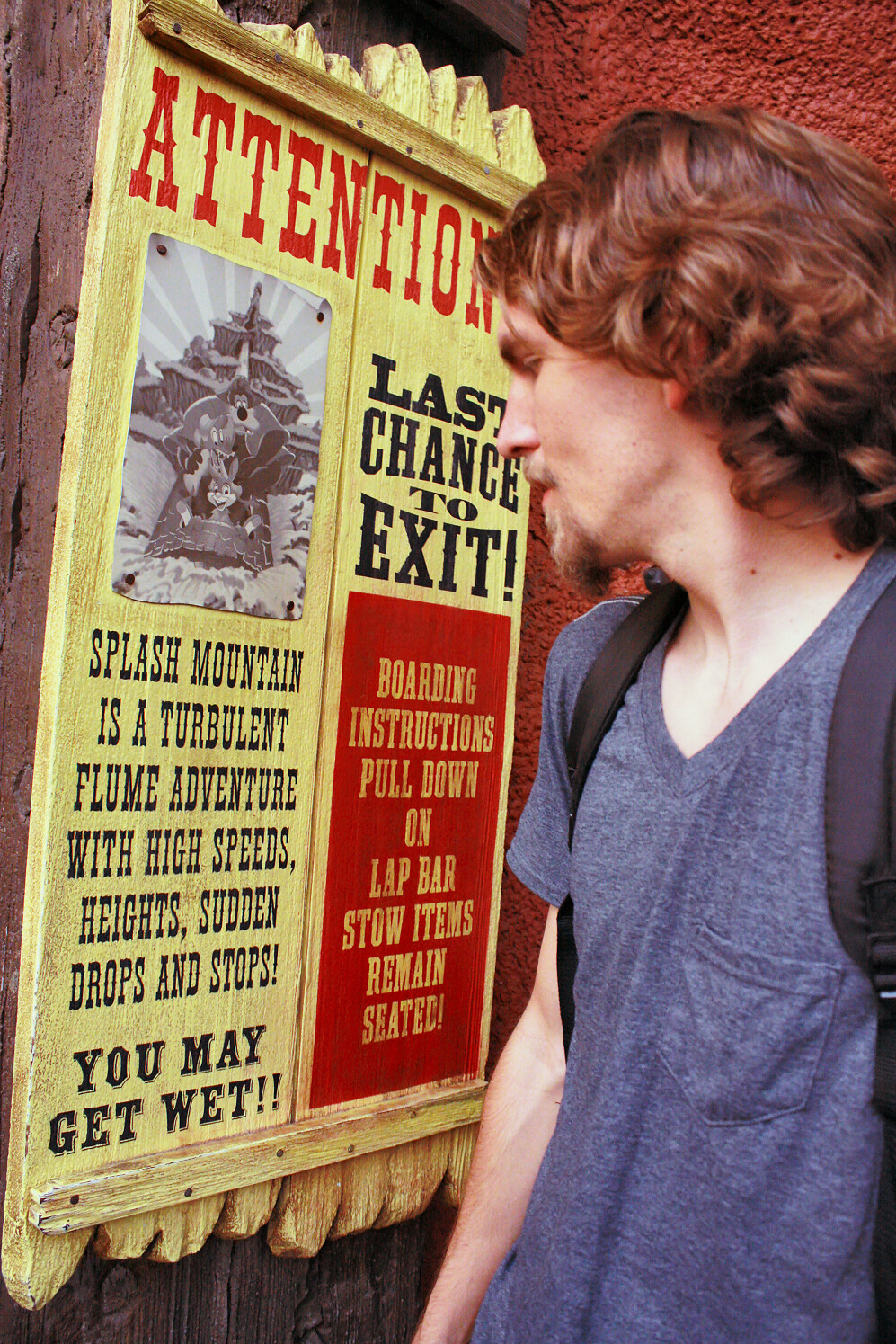The image depicts a young man with long, curly brown hair and a goatee, wearing a gray t-shirt and carrying a black backpack, with visible straps over his shoulders. He stands in front of a reddish rock-like wall, gazing at a wooden sign at an amusement park. The sign, made of wood and painted yellow with red lettering that reads "ATTENTION! Last chance to exit," informs visitors that "Splash Mountain is a turbulent flume adventure with high speeds, heights, sudden drops, and stops. You may get wet." The right side of the sign provides boarding instructions: "Pull down on lap bar. Stow items. Remain seated." Adjacent to the text, there is a cartoon depiction of characters on a raft coming down a mountain, emphasizing the adventurous nature of the ride.